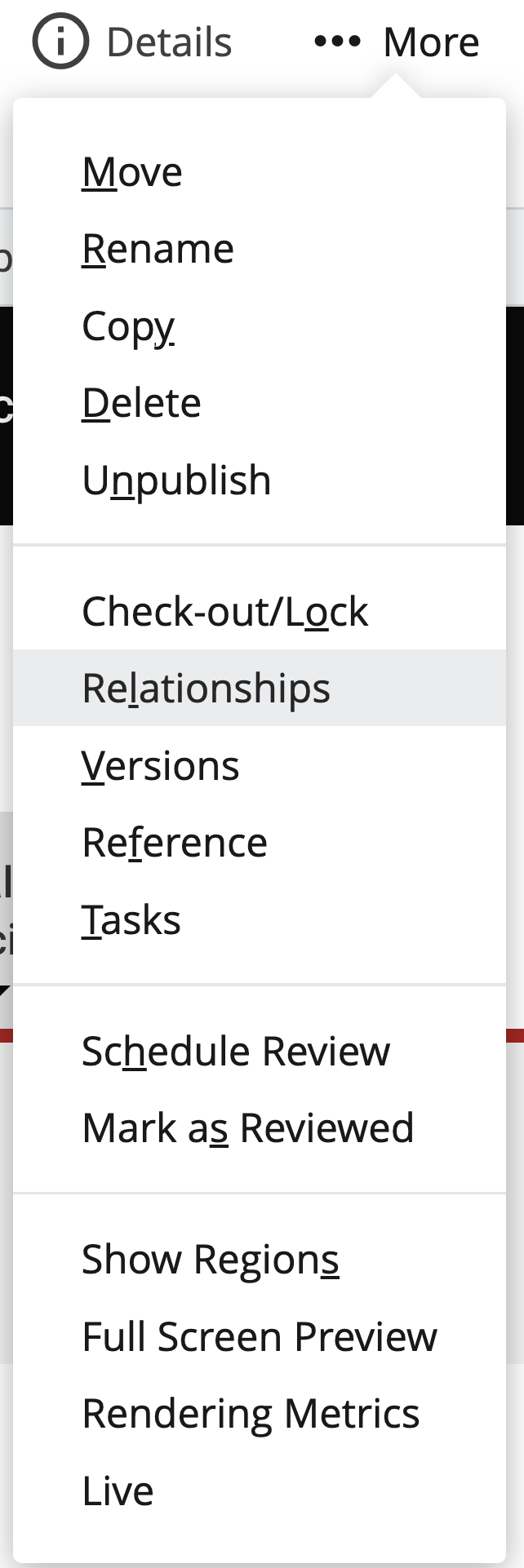The image depicts a vertical, rectangular drop-down list overlaid on a webpage. The drop-down list has a white background, with dark gray text, and several options listed. At the very top of the list, an icon resembling an eye encircled is placed next to the word "Details," followed by three vertical dots and the word "More" to the right. It appears that the "More" option has been clicked, revealing the drop-down menu.

The menu contains a series of options: "Move," "Rename," "Copy," "Delete," "Unpublish," "Checkout/Lock," "Relationships" (highlighted with a gray ribbon), "Versions," "Reference," "Tasks," "Schedule Review," "Mark as Reviewed," "Show Regions," "Full Screen Preview," "Rendering Metrics," and "Live."

In the background, the actual webpage is visible. The top part of the webpage has a white background, followed by a thick blue band that might appear black due to lighting or resolution. The remainder of the webpage predominantly features a white background. The detailed contrast between the interface elements of the drop-down list and the webpage provides a clear view of both components, highlighting the functionality and design features.